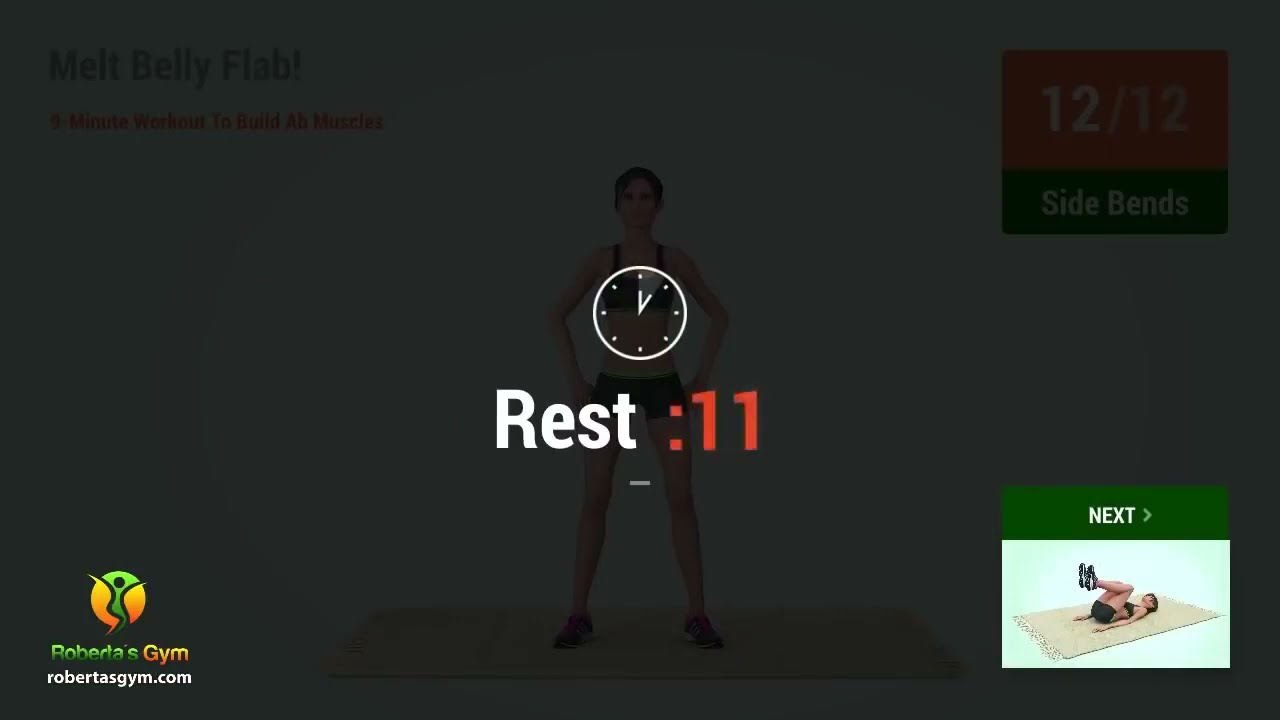The image is a screen capture from the website robertasgym.com, featuring an interactive exercise tutorial overlaid with a semi-transparent black filter. At the center, a woman, possibly 3D rendered, stands upright on a tan mat wearing a black sports bra and black pants against a white background. Text above her reads "Melt Belly Flab," and on the right, it indicates that "12 of 12 Side Bends" have been completed. A white clock icon in the center shows "Rest: 11 seconds." In the bottom left corner, the yellow and green logo of Roberta's Gym is visible along with the website URL. The bottom right corner displays a thumbnail of a photorealistic woman performing a workout pose, with a green box above it stating "Next."